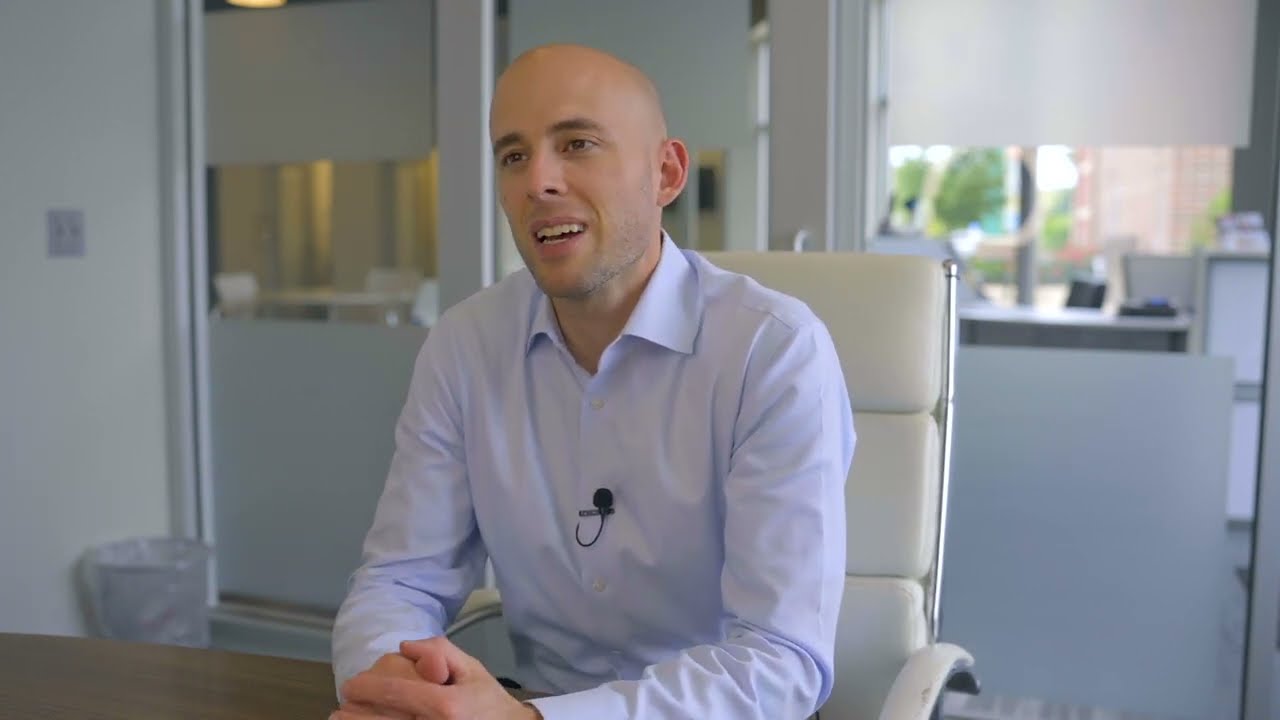In this detailed office scene, a bald man is captured sitting slightly left of center in a white high-back office chair with white armrests. He is wearing a light blue button-up shirt with the top button unbuttoned and has a small black microphone clipped to the center of his shirt just above his chest. With a thoughtful expression, his mouth is open, visibly showing his top teeth and a hint of his bottom row, suggesting he is engaged in an ongoing conversation, likely an interview.

His brown eyes are open, directed towards the left, focusing just past the shoulder of the camera. His hands are clasped together and resting on a dark brown wooden table in front of him. The background, which is slightly blurred, reveals the office setting with a desk accompanied by a black phone and a filing cabinet. There is a window that brings soft light into the room, and a white table on the left side. In the bottom left corner of the image sits a gray trash can covered with a plastic bag, placed against a white wall that features a double light switch.